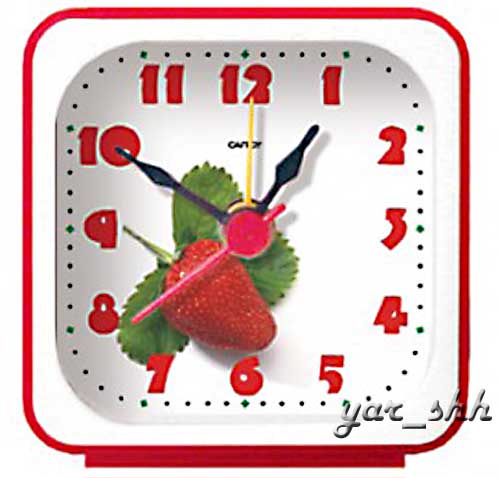This image features a unique analog clock set against a detailed backdrop. The clock itself is framed within a red square with rounded corners, containing a white clock face that also has rounded edges. Surrounding the clock are small black dots marking the minutes, with larger green squares indicating the hours. The numbers on the clock face are thick, bold, and colored red, running sequentially from 12 at the top to 6 at the bottom.

At the center of the clock, it reads "CAT" in black text, though partially cut off. The clock hands consist of three distinctive colors: a black hour hand pointing towards 1, a black minute hand indicating 10 (representing 1250), and two seconds hands—one yellow pointing at 12 and another red slightly below the 8, possibly indicating milliseconds.

The background to the bottom-left features a vibrant strawberry with three green leaves—two on the right and one on the left—and a green stem pointing to the left. In the bottom right corner of the image, partial text reads "Y-A" and possibly "T," followed by an underscore and "SHH."